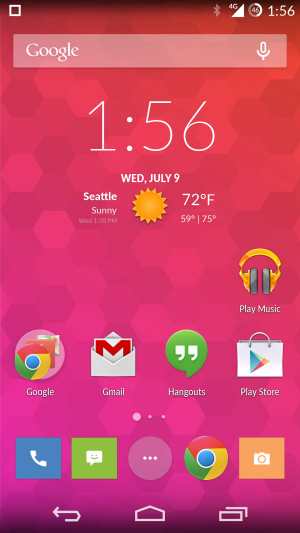The image depicts a smartphone interface in portrait mode. At the top, there's a search bar labeled "Google Enlight" with a microphone icon to the right. The background of the phone is a gradient transitioning from reddish at the top to purplish at the bottom, featuring a honeycomb pattern.

Displayed prominently in white text is "1:56" with smaller text below reading "Wednesday, July 9th". It shows localized information: "Seattle, Sunny, Wednesday 1:50 PM" along with a yellow sun icon. The weather details, "72°F, 59°F/75°F", are positioned to the right of the sun icon.

Several app icons are arranged below the time and weather information. On the right, there's a yellow headphone icon labeled "Play Music". To the left of it are a series of icons: the Google icon, Gmail, and a green speech bubble with white quotations representing Hangouts. Next to Hangouts is a white bag with a colorful arrow, denoting the Play Store.

Further down, there are more app icons in a horizontal row: a blue icon with a phone, a green icon featuring a happy face inside a speech bubble, a clear button with three white dots, the Chrome icon, and an orange icon with a white camera.

At the very bottom, the screen displays navigational symbols, completing the detailed phone interface.